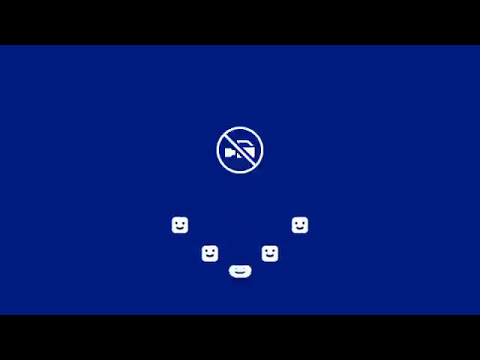The image resembles a computer error screen, specifically evoking the notorious Microsoft blue screen of death, but with a playful twist. Dominated by a solid blue center framed by thick black bars at the top and bottom, it features a prominent "no camera" symbol—a vintage handheld video camera inside a circle with a slash through it—indicating a prohibition on cameras. Directly beneath this symbol is a playful arrangement of smiley faces in white. These faces form a V shape: two squares with smiley faces on either side slanting upward, and a central elongated smiley face at the bottom, collectively resembling a large, smiling face. The minimalist color scheme of blue, black, and white, and the absence of text, give it the feel of a warning or error message, possibly captured from a PlayStation console.